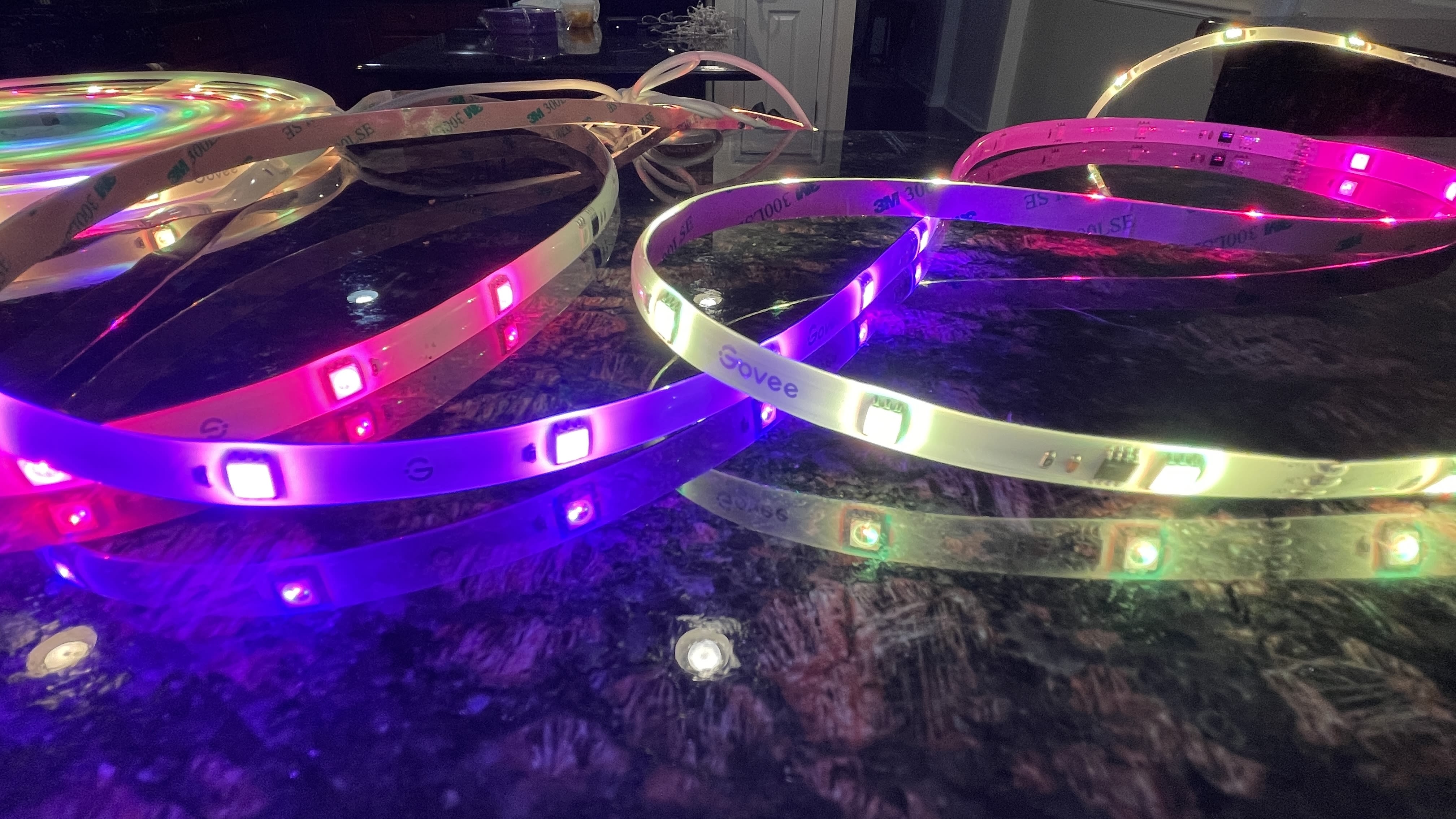In the photograph, several coiled, LED light strips from the brand Govee are laid out on a patterned marble tabletop that features shades of brown and black. You can see the reflection of the lit LEDs on the countertop, with vibrant colors including purple, pink, green, and a bluish-purple. The strips are labeled with the brand name Govee and have a sticky backing provided by 3M, specifically labeled 3M 300L. To the left of the coiled strips, an uncut string of LED lights extends out. Additionally, there is a circular disc-like object in the top left corner of the image, illuminated with pink, green, and blue colors. In the background, another marble countertop is visible, along with a white-painted open door leading to a hall. The overall setting hints at a kitchen environment.